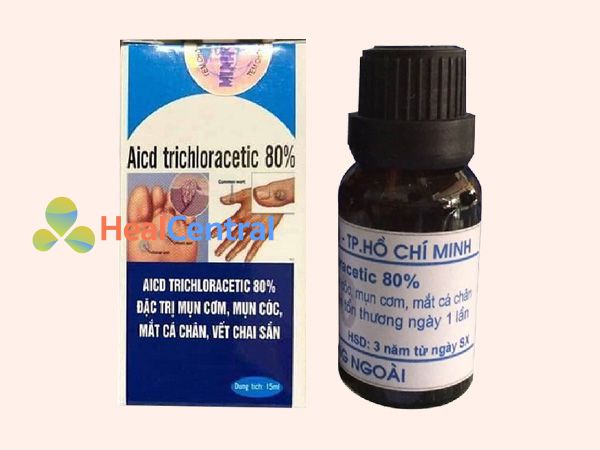The image features a square box with a very faint pink background, focusing on two main components: a product box and the corresponding medication bottle. The box prominently displays the text "Acid Trichlorate 80%," along with some additional wording in an Asian language, likely Thai. "Heal Central" and a logo consisting of a three-leaf clover with green, blue, and yellow leaves are also visible on the box. The box is predominantly white with blue accents and has a dark blue bottom. A small illustration of a foot and a hand appears on the front, hinting that the product is intended for treating warts on these areas.

Next to the box is the medication bottle, which is an opaque dark brown with a large black screw-top stopper. The bottle features a white label with blue text, including "Acid Trichlorate 80%" and more writing in Thai. The setting of the image suggests that it is meant to inform viewers about this wart treatment product, emphasizing its availability for purchase.